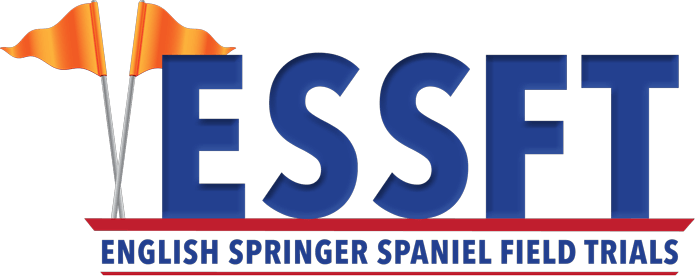The image features a distinctive logo set against a plain white background. Dominating the top left corner, two diagonal gray poles intersect, each adorned with a flying orange flag. At the center of the image, large, bold, blue letters spell out "ESSFT." Directly beneath this, a thin red line and bold blue text in all caps read "ENGLISH SPRINGER SPANIEL FIELD TRIALS," further defined by another horizontal red line below. The overall composition lacks additional elements such as animals, people, or extra text, focusing entirely on the blue and red logo elements and the orange flags.